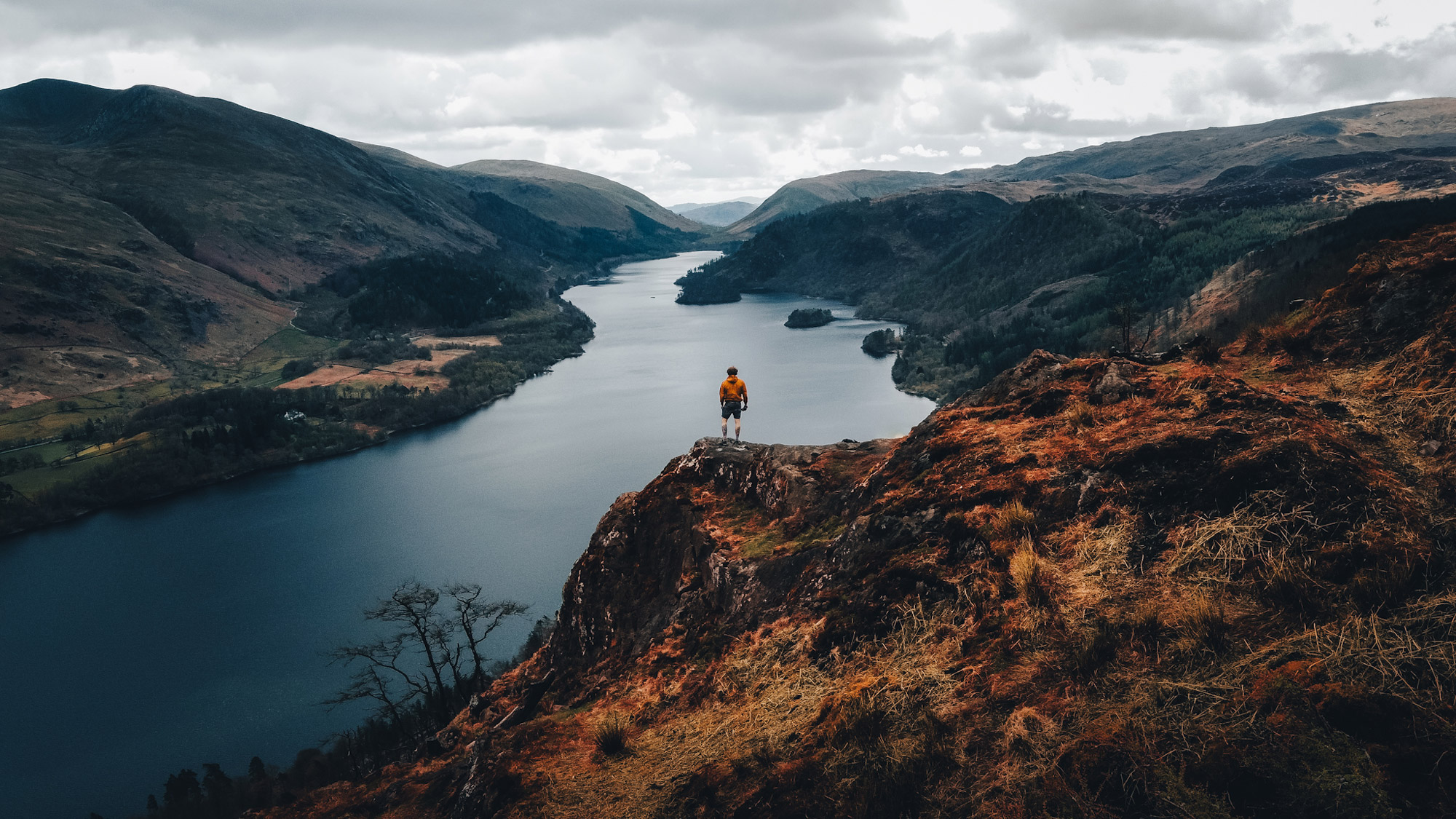In this captivating landscape image, a man stands on a rugged canyon overlook, with a winding river creating a charming pathway from the bottom left corner to the center of the frame. He is dressed in a yellow coat and black shorts, his dark hair contrasting with the overcast sky. The river below, with its dark waters reflecting sunlight in the middle, flows smoothly between brownish, reddish, and tan rocky formations that dominate the foreground. On the left, mountains rise majestically while rough canyons and rocky terrain make up the middle of the image, where the man stands. The sky is covered with gray and black clouds, adding a dramatic backdrop to the scene. The photo, likely taken from afar with a telescopic lens, captures a serene yet powerful landscape with the man appearing small amidst nature’s vast beauty.